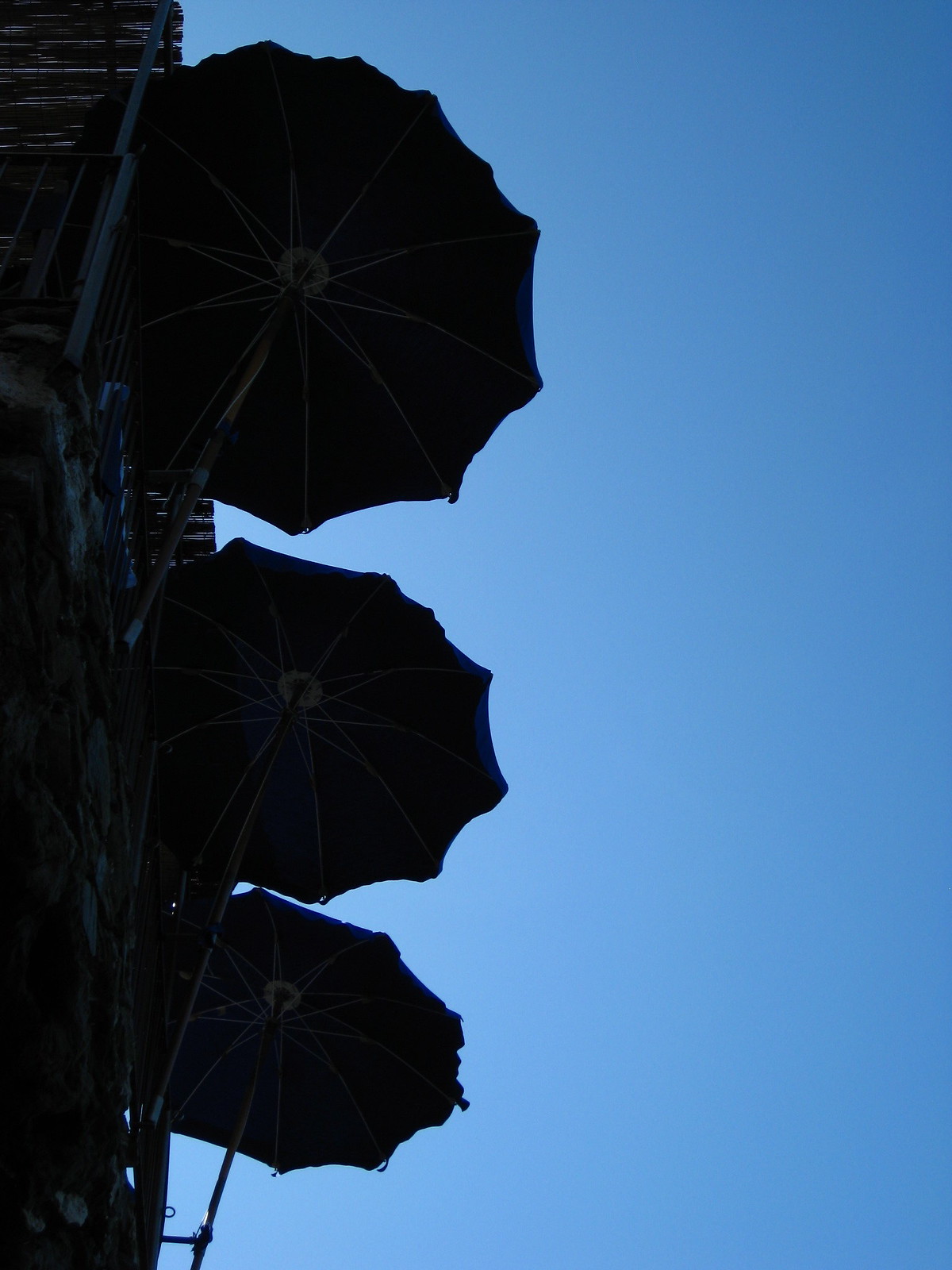This color photograph captures an upward view of three dark navy umbrellas mounted on the edge of a rock deck or balcony structure. Each umbrella is supported by a metal bracket and features flared metal pieces extending to its edges, silhouetted against a pristine, cloudless blue sky. The umbrellas, arranged vertically on the left-hand side of the image, appear to be stacked with the smallest at the bottom, the medium one in the middle, and the largest on top. Behind them is a wooden roof and a dark-colored metal railing in the top left corner, adding to the intricate composition. The overall scene evokes a sense of delicate antiquity and serene beauty, highlighted by the warm hues of early morning or late evening light.